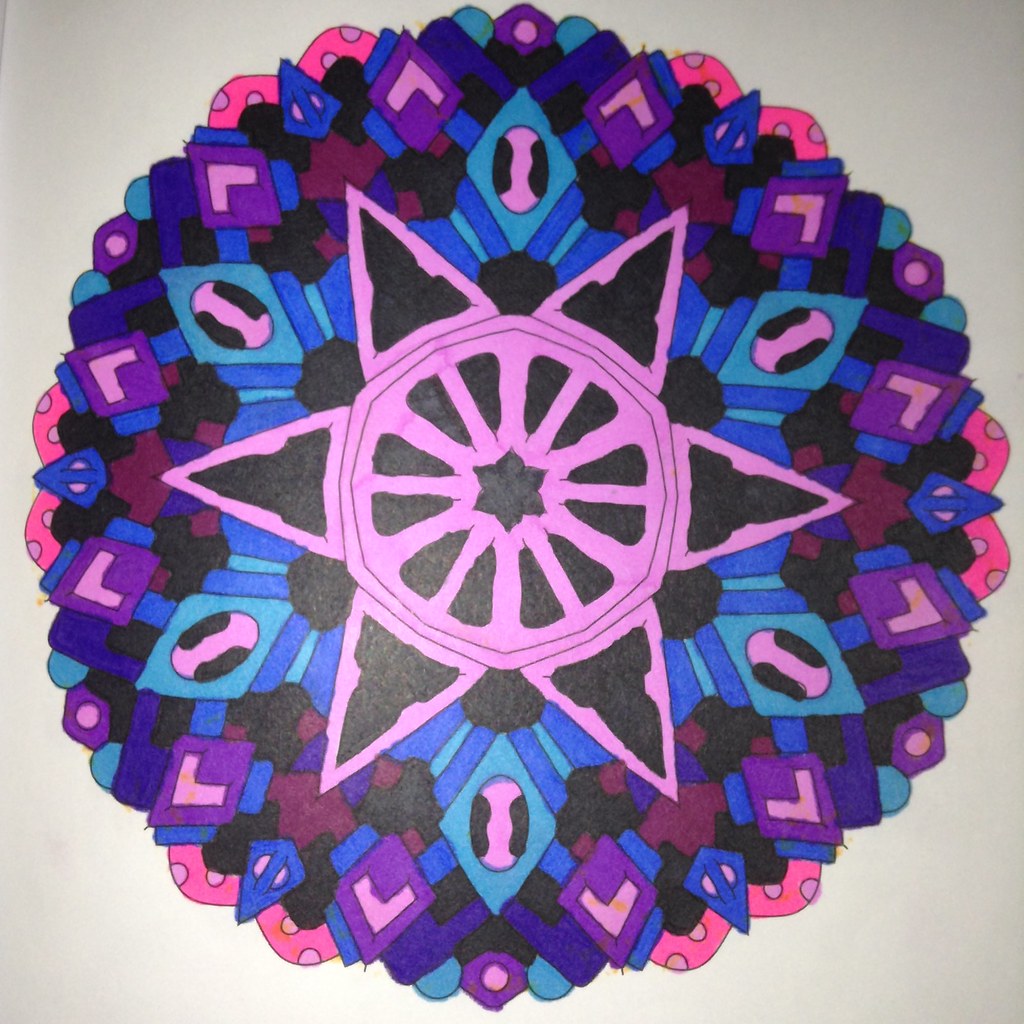This image captures a square photograph of a vibrantly colored mandala set against a white or off-white background. The intricate mandala, which appears hand-drawn or possibly computer-generated, showcases a rich palette of pinks, blues, purples, magenta, dark red, and black. At its core, it features two interlocking triangles resembling the Star of David, with one triangle rotated so the stars align horizontally. Surrounding the central motif are concentric rings adorned with evenly spaced black shapes, creating a harmonious and symmetrical design. Every section of the mandala is meticulously filled with color, leaving no white spaces within the intricate patterns. The precise detailing suggests careful craftsmanship, possibly executed with markers.